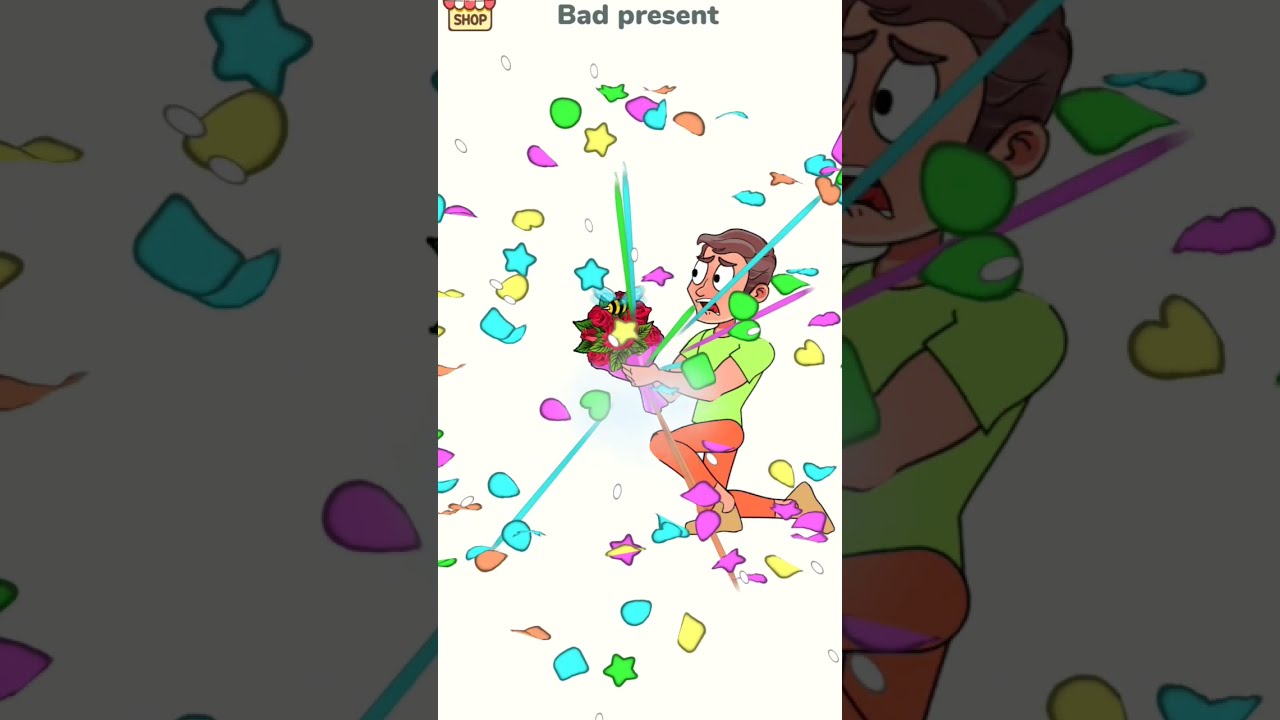In this vibrant, cartoon-style image set against a completely white background, a startled light-skinned man with wide eyes and a perplexed mouth expression is the central focus. He has short dark brown hair, brown eyebrows, and large white eyes with black pupils. The man, who is kneeling on one knee with the other knee bent and foot planted on the ground, is dressed in a bright lime green shirt, orange pants, and light beige-brown shoes. Clutched in both his hands is a bouquet of red roses, from which an explosion of colorful confetti bursts forth, including blue stars, yellow blobs, green ovals, hearts, circles, and other vibrant shapes surrounding him. At the top of the image, in bold black letters on a white background, the caption reads "Bad Present." To the left, "Shop" is written in black letters with small dots above it. The image is framed by dimmed, zoomed-in rectangular sections of the central cartoon, which extend across the left and right sides, creating a cohesive yet exaggerated effect that highlights the chaotic energy of the scene.